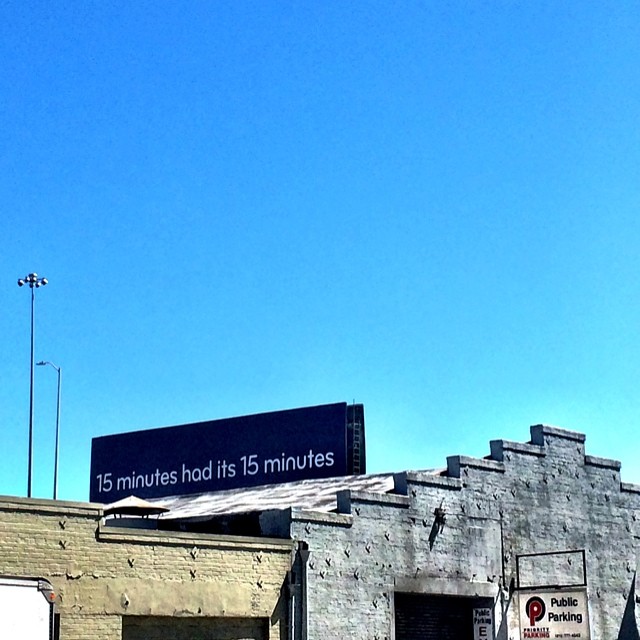The photograph captures a striking urban scene dominated by a large, rectangular blue billboard mounted atop a meticulously geometric stone building. The billboard, in a vivid blue shade, boldly displays white text proclaiming, "15 minutes had its 15 minutes." The structure hosting this advertisement is a light gray stone building, characterized by a terrace-like pattern of intersecting rectangles that ascend towards its roof.

Adjacent to this gray stone building is another structure made of light tan or light brown colored stone bricks, adding a subtle contrast to the scene. The backdrop features a vibrant blue sky that transitions from a lightish blue-teal color near the horizon to a brighter, more traditional blue towards the top of the image. The clarity and brightness of the sky enhance the overall vibrancy of the photograph.

To the left of the billboard, two slender metal street lamp poles ascend, contributing to the urban aesthetic. Additionally, a white rectangular public parking sign is visible at the bottom right corner of the image, hanging from the gray stone building, providing a practical detail to this urban landscape.